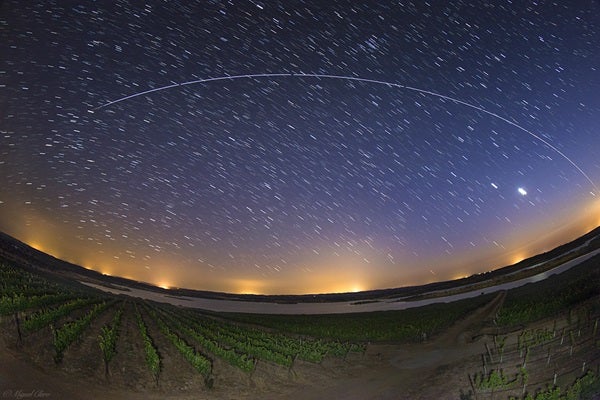This captivating photo, captured with a fisheye or 360-degree lens, presents a half-arc panoramic view of a star-studded night sky above a sprawling landscape. The sky, rich with a vast number of stars, shows them as small, blurred lines, hinting at a long exposure shot. Dominating the celestial field is a distinctive white line, possibly a shooting star, curving along the same arc as the overall photo. Below this celestial display, the landscape features a waterway and rows of plants, possibly cornfields, intersected by dirt roads. The horizon is lined with yellow lights, contrasting subtly with the dark expanse of the night. Despite some blur in the image quality, the intricate details of the stars, fields, and lights create a mesmerizing scene.